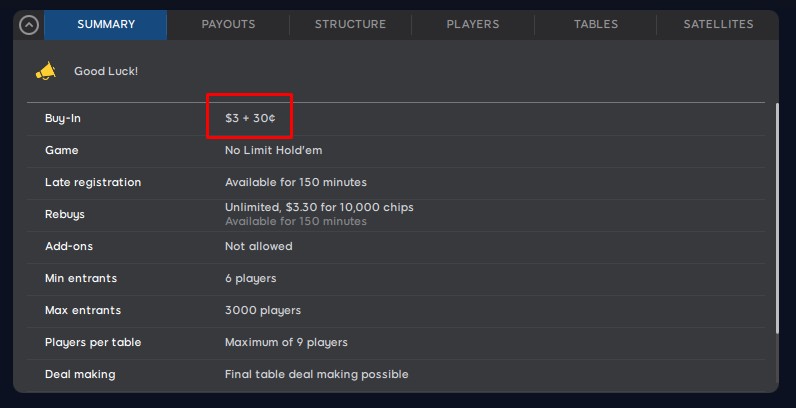This is a screenshot of a buy-in summary for an online poker platform, meticulously cropped to focus on the essential details. The background of the interface features a dark blue color scheme, providing a sleek and professional aesthetic. Dominating the center of the image is a large, grey overlay screen, which stands out prominently against the darker background.

At the top left corner of this overlay, a navigation bar is visible, listing several tabs: "Summary," "Payouts," "Structure," "Players," "Tables," and "Satellites." In the extreme top-left corner, there is an icon of an upward-pointing arrow inside a circle, suggesting that the menu can be collapsed or minimized.

Directly below the "Summary" tab, on the left side of the screen, a megaphone icon is shown, accompanied by the phrase "Good Luck" displayed in white font, adding a touch of encouragement for the players.

On the right side of the screen below this section, there is a detailed list containing various pieces of information about the tournament. The list starts with the buy-in details, clearly stating "$3.00 + $0.30" next to a red box that has been edited onto the screen to highlight the buy-in amount.

Further down, additional key details are provided: the game type is specified as "No Limit Hold'em," and late registration is noted to be available for 150 minutes. The option for unlimited rebuys is also mentioned, along with other relevant information about the tournament structure and rules.

Overall, this well-organized screenshot offers a comprehensive summary of the buy-in and related details for participants in the online poker event.